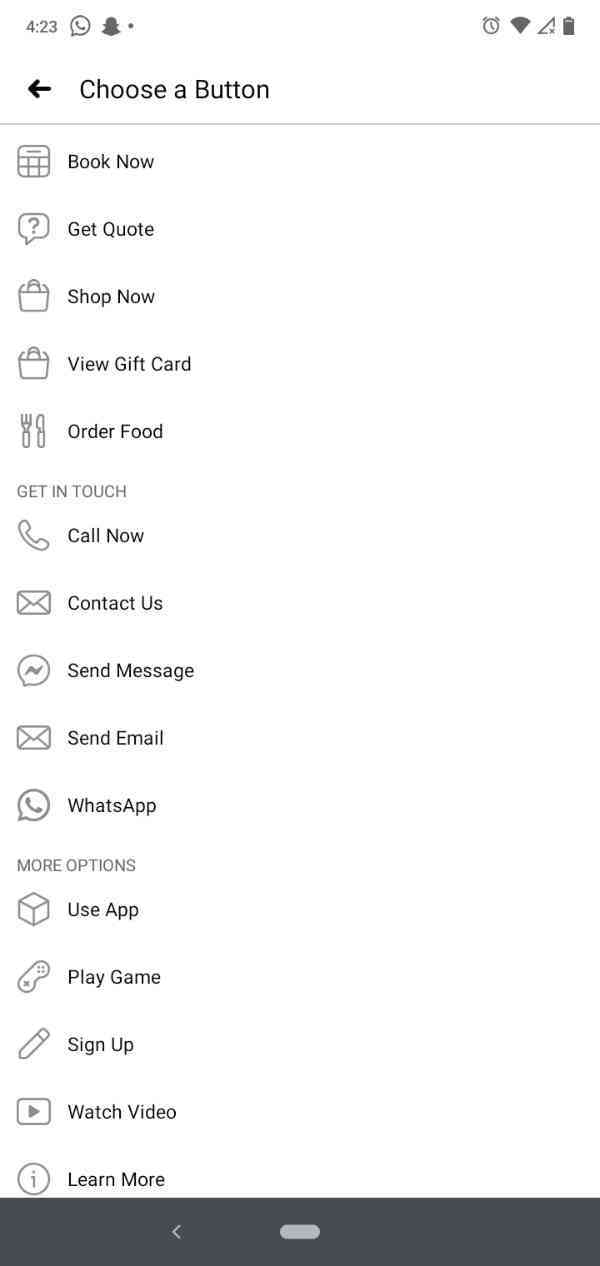This image is a screenshot taken from a mobile device, likely an Android based on the presence of navigation buttons at the bottom, including a back arrow. The screen showcases a settings or options menu with a white background.

At the top, there's a back arrow icon followed by the text "Choose a button." Below this header, the screen displays several icons paired with corresponding text labels for various actions:

1. **Calendar Icon:** "Book Now"
2. **Question Mark Icon:** "Get Quote"
3. **Shopping Bag Icon:** "Shop Now"
4. **Another Shopping Bag Icon:** "View Gift Card"
5. **Knife and Fork Icon:** "Order Food"
6. **Phone Icon:** "Call Now"
7. **Envelope Icon:** "Contact Us"
8. **Speech Bubble with Squiggly Line Icon:** "Send Message"
9. **Another Envelope Icon:** "Send Email"
10. **WhatsApp Icon:** Displaying further options

The menu appears to provide a variety of quick access options for different services or actions, making it a comprehensive and user-friendly interface.